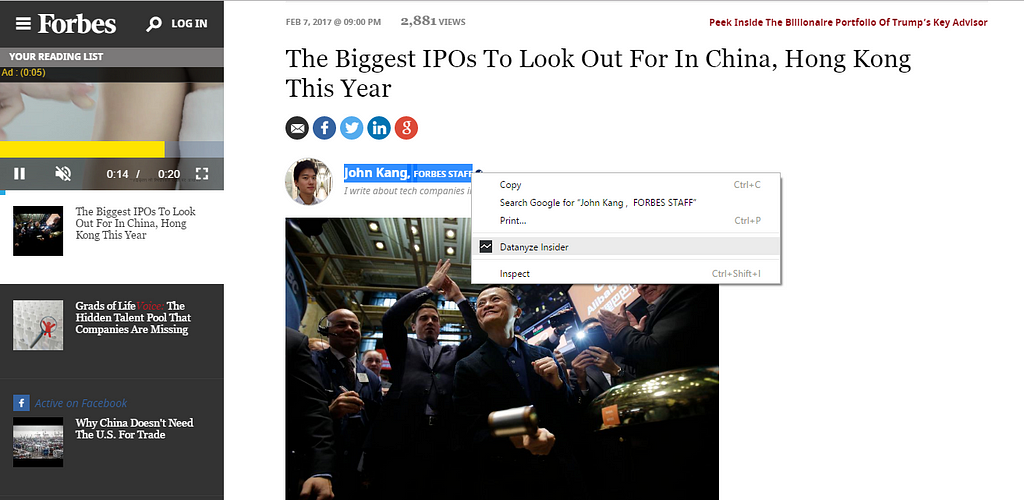**Detailed Caption:**

The image showcases a section of a website, specifically a Forbes article page.

### Left Panel:
At the top, there are two square icons:
1. The top-most square contains three white horizontal lines stacked vertically, indicating a menu.
2. Adjacent to this icon is the Forbes logo, prominently displayed with a capital "F".

Next, there is a magnifying glass icon symbolizing the search function, followed by the word "LOGIN" in capital letters.

Below this header, the background shifts to a light to medium gray. Here, it displays "Your Reading List" in white text, and beneath it, there is an "Add" button printed in gold. Parenthetically, it notes "(0.05)", alongside a small graphic element.

Continuing downwards, a yellow banner appears, overlaid with a darker gray banner containing media control icons, including "pause" and "volume". It shows a timeline with the values "0.14 / 0.20". Below these controls, there's a small white space presumably reserved for text.

Further down, a headline reads: "The Biggest IPOs to Look Out for in China, Hong Kong This Year."

Another square box appears in light black, featuring:
1. "Grads of Life" in white text.
2. "Voices" in red text.
3. The sub-heading: "The Hidden Talent Pool That Companies Are Missing."

### Additional Topics:
- "Active on Facebook."
- A headline: "Why China Doesn’t Need the US for Trade."

### Center Panel (Main Article):
The main portion of the page features the article itself. It also begins with the headline: "The Biggest IPOs to Look Out for in China, Hong Kong This Year."

Underneath, there are circular social media icons for:
1. Email (represented by an envelope).
2. Facebook
3. Instagram
4. Twitter
5. LinkedIn
6. Energy (possibly indicating an RSS feed or similar icon).

The article is authored by John King, indicated by "John King, Forbes Staff," alongside his profile image.

A graphic at the bottom shows various people in an office setting, adding a visual element to the article's topic.